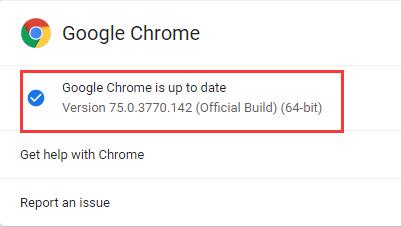The image showcases a Google Chrome update notification. At the top, it states "Google Chrome is up to date," followed by the version number "75.0.3770.142." The notification specifies that it is the "Official Build" and "64-bit." Below this information, there are two options: "Get help with Chrome" and "Report an issue." All this text is contained within a gray box, which is set against a white background. Additionally, a thick red border surrounds the entire Google Chrome section.